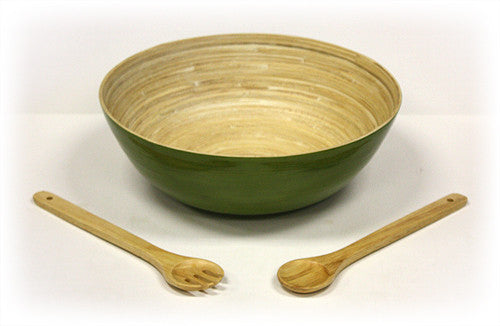The image features a handmade wooden bowl, accompanied by a matching wooden fork and spoon, arranged on a light beige or white surface. The bowl is positioned centrally with a glossy green exterior and an intricately exposed wood grain interior, showcasing various shades of brown. The wooden salad fork and spoon, both light brown with simple designs, are placed diagonally in front of the bowl, with the fork on the left and the spoon on the right, each ending near the bottom center of the image. The utensils also feature small holes at the end of their handles, likely for hanging. The image background fades to white around the edges, suggesting it may have been taken in a light box or edited to emphasize the objects.